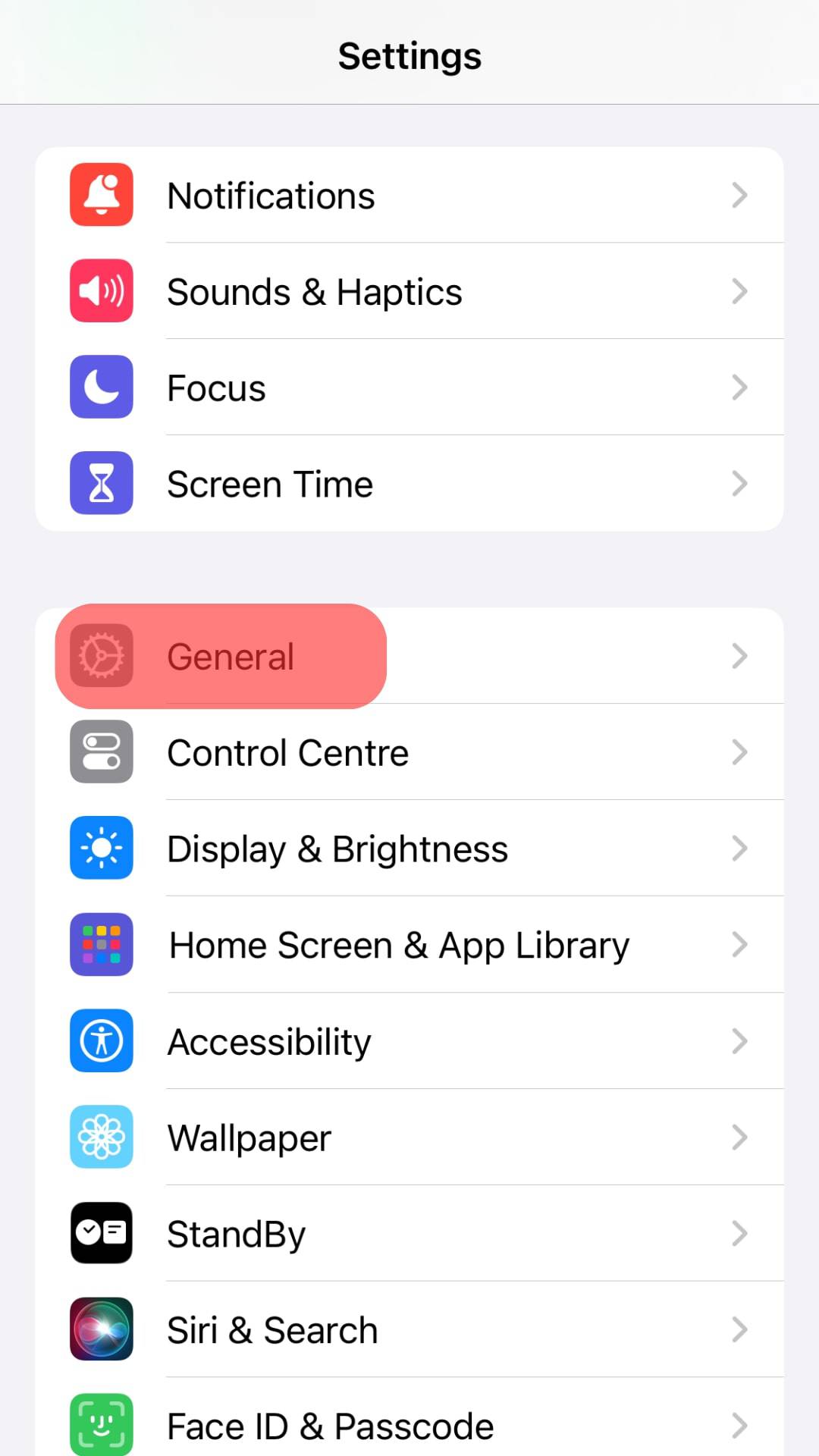This image is a screenshot taken from a phone, displaying the "Settings" menu against a white background. The primary "Settings" header is followed sequentially by various options each accompanied by distinct icons:
 
1. **Notifications** - Illustrated with a small bell icon.
2. **Sounds & Haptics** - Represented by a little speaker icon.
3. **Focus** - Shown with a crescent moon icon.
4. **Screen Time** - Depicted with an hourglass icon.
5. **General** - Highlighted within a red box featuring red text and a steering wheel icon.
6. **Control Center** - Marked by an icon with various buttons.
7. **Display & Brightness** - Identified with a sun icon emitting rays.
8. **Home Screen & App Library** - Displayed in a blue box containing colorful squares.
9. **Accessibility** - Indicated by a blue box with a round circle containing a body with extended arms.
10. **Wallpaper** - Signified by an aqua box with a daisy-like flower icon.
11. **Standby** - Encased in a black box with a circle and a checkmark, followed by another box with small text.
12. **Siri & Search** - Featured in a black box with multifaceted colors.
13. **Face ID & Passcode** - Encased in a green box with a simplistic face icon.

This detailed cascade of settings options provides a comprehensive view of the user’s customizable features on the device.